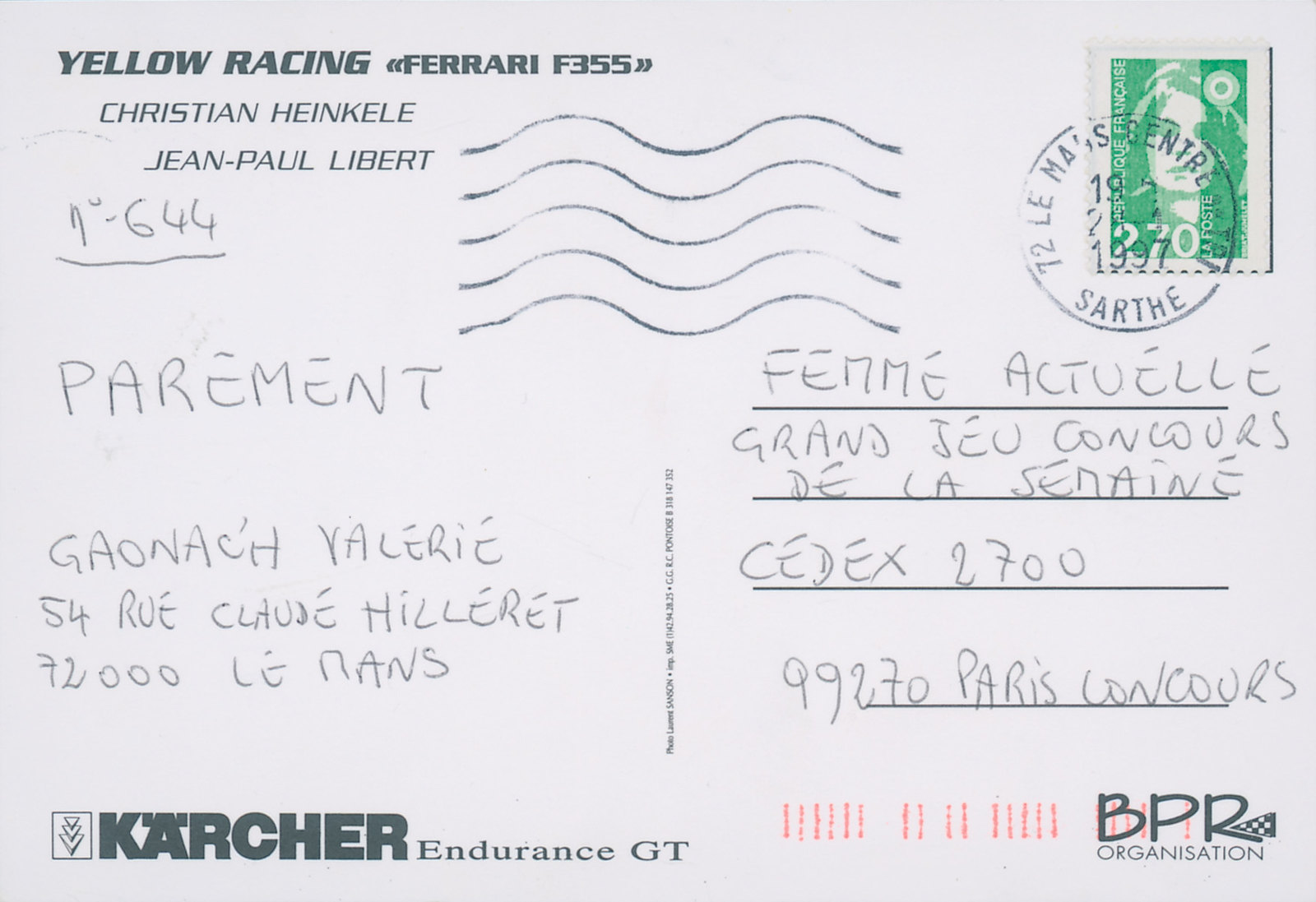The image captures a detailed close-up of a postcard, with various elements that fill the entirety of the frame. Dominating the top left section, the text reads "Yellow Racing Ferrari F355, Christian Heinkel, Jean-Paul Libert" typed prominently. Below, handwritten in French, it says "1/644, Parament, Guanach, Ya, Valerie, 54, Rue, Clos, Hilleret, 7200, Le Mans," suggesting the recipient's address. In the top right corner, there's a green and white stamp featuring a female's face, along with a clearly visible postmark. The left side of the card includes "Femme Actuelle, Grand Loup, Concours de la Semaine, CEDEX 2700, 99270, Paris Concours," likely the sender's address or a reference to a contest. The postcard’s design includes a combination of typed and handwritten text in black ink, against a background featuring whites, greens, and reds. A barcode is seen at the bottom, aligning with the format typical of address sides of postcards.